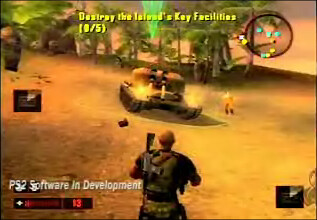This detailed image is a screenshot from a third-person shooting game, reminiscent of PS2-era graphics. Dominating the top portion of the screen is yellow text reading "Desert Ray, the island's key facilities," followed by "0/5." Positioned slightly to the right of this is a black circle containing various blue and yellow squares, with one orange square below them. The background showcases a vibrant palette of purples, oranges, and yellows, transitioning into sparse trees and rocky terrain on the left, and denser vegetation toward the center-right. Prominently in the middle foreground is an upside-down, diamond-like peak resembling an icicle.

Directly below this, the sandy desert ground is occupied by an army tank oriented towards the viewer, its brown turrets actively firing, indicated by visible light flashes. To the forefront stands a soldier, seen from behind, wearing a green outfit complete with a hat, jacket, and pants. He has a rifle strapped over his left shoulder, and the low-poly graphics attribute a retro charm to his appearance. In the bottom left corner, white text states, "PS2 Software and Development," accompanied by a rectangular red health bar and a small square displaying the number three. Sparse trees and a rocky outcrop bolster the setting’s rugged aesthetic, emphasizing the game's intense, strategic environment.